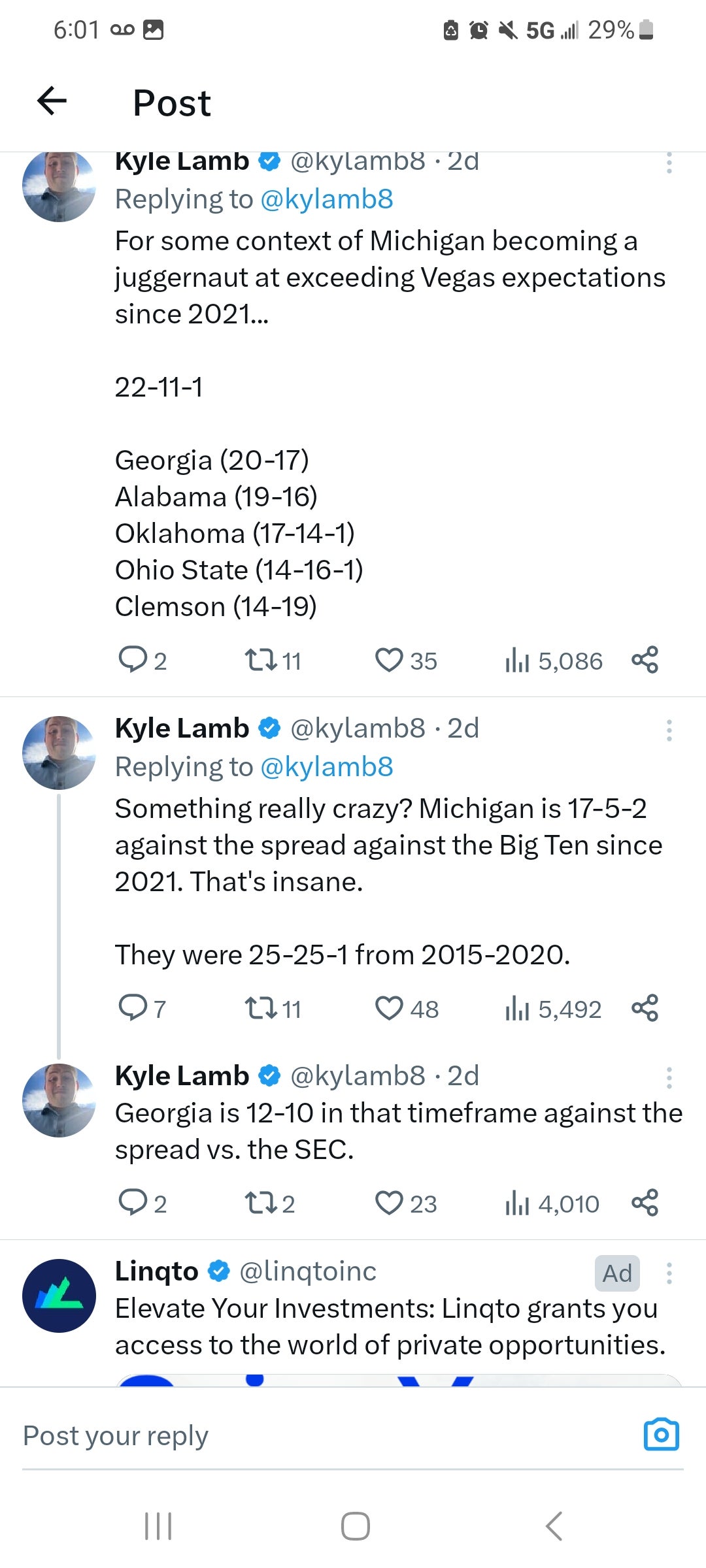This is a screenshot of a Twitter thread posted by Kyle Lamb (@KyleLamb8) two days ago. The conversation captures Kyle's analysis of the Michigan football team's performance against Vegas expectations since 2021. 

The first tweet in the thread sets the context by comparing Michigan's record to other notable college football teams:
- Michigan: 22-11-1
- Georgia: 20-17
- Alabama: 19-16
- Oklahoma: 17-14-1
- Ohio State: 14-16-1
- Clemson: 14-19

The post has two comments, 11 retweets, 35 likes, and 5,086 views.

The second tweet in the thread highlights Michigan's impressive performance against the spread in Big Ten games since 2021:
- Record since 2021: 17-5-2
- Record from 2015 to 2020: 25-25-1

This tweet has seven comments, 11 retweets, 48 likes, and 5,492 views.

The final tweet provides a comparison to Georgia's performance against the spread in SEC games over the same time frame:
- Georgia's record: 12-10

It has two comments, two retweets, 23 likes, 4,010 views, and includes a promotional link to "Linqto Inc," encouraging users to elevate their investments by accessing private opportunities. The link is labeled as a promotional ad.